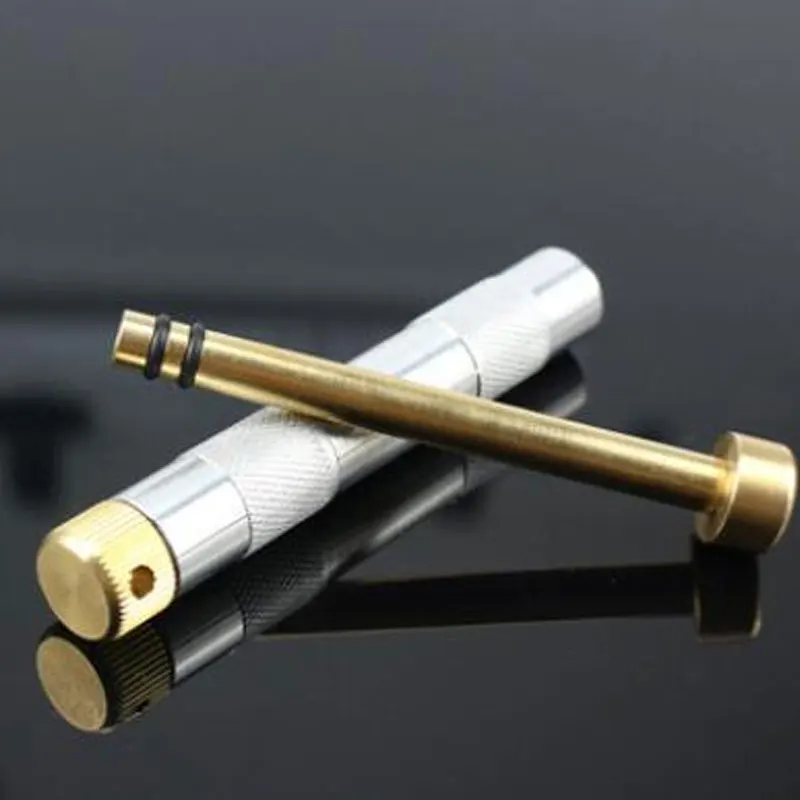Displayed on a black, shiny, reflective surface, the image showcases a peculiar handheld tool whose exact purpose is unclear. The primary component resembles a hammer, laying with its brass head touching the ground and its handle extending upwards. This handle features two black rubber bands near one end. Underneath the hammer part, there is a wider stainless steel cylinder, which also acts as part of the device. This cylinder includes two white bands with a textured grip and ends with a golden, twistable cap with a single hole, possibly designed for a key wrench. Overlapping the cylinder, a secondary component made entirely of brass, possibly hollow, sits diagonally. This brass piece seemingly has no evident attachment point but might screw onto the other part. The entire setup hints at some form of nozzle-like mechanism but leaves its exact function open to interpretation.